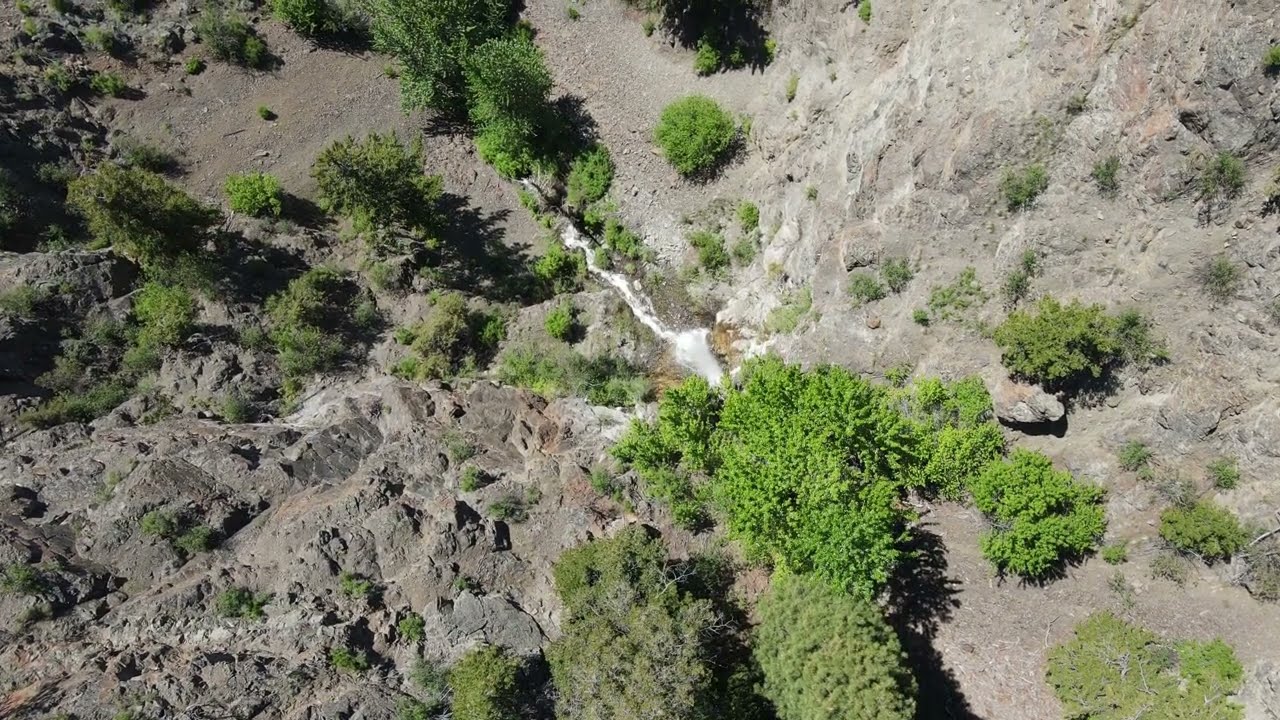The photograph, taken outdoors during the daytime from an elevated perspective, vividly captures a steep hillside or canyon plunging towards a rocky bottom. The terrain is predominantly barren, composed of dark gray and reddish stones, with no grass, only sparse vegetation clinging to the rugged slopes. A sinuous, white-foamy stream runs through the center of the canyon floor, bordered by spotty patches of vibrant green. These patches include bushes, small trees, and shrubbery, which are densest where the water flows. The natural light enhances the stark contrast between the arid, stone-laden slopes and the lush greenery at the bottom, showcasing the dynamic interplay of colors—gray, green, white, and brown. The image, clear and highly detailed thanks to the bright daylight, highlights the raw, untouched beauty of this remote, uninhabited landscape.